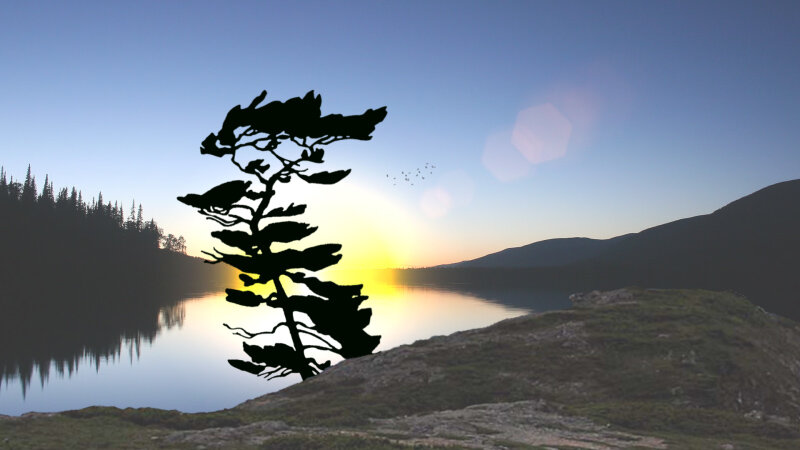The image depicts a tranquil nature scene at either sunset or sunrise, featuring a body of water bordered by moss-covered hills and silhouetted pine trees in the background. The central focus is a striking, dark silhouette of a plant, standing prominently in the foreground, seemingly swaying. This plant is brilliantly highlighted by the golden yellow glow of the sun at the horizon, casting a serene and reflective ambiance over the water. The composition is rendered mostly in dark silhouettes, accentuating the mystical and abstract quality of the scene, with a soft reflection of the trees and hills on the water's surface. Subtle details include rocky land in the foreground, a blue sky with shimmering light cells, and a distant, faint flock of birds.